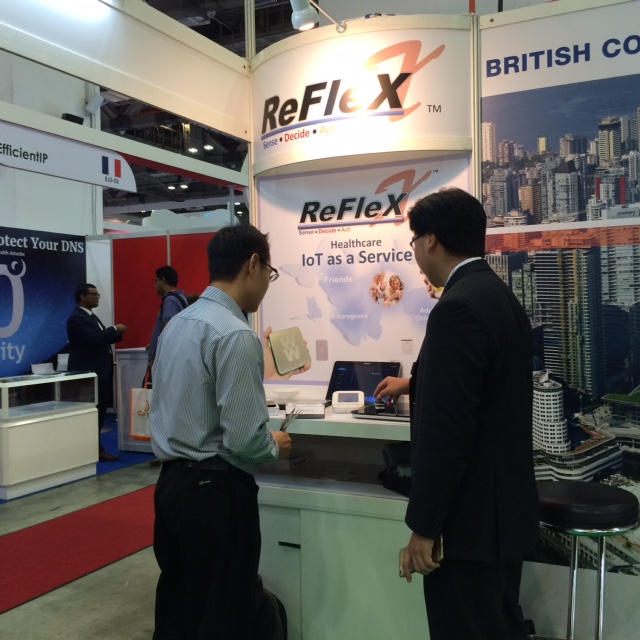In a bustling exhibition setting, two men stand engaged before a sleek, modern kiosk labeled "Reflex." The prominent sign features the word "Reflex" in large black letters, with a distinct orange 'E' against a white curved backdrop. Beneath this title, the display reads "Healthcare IoT as a Service," and the module is flanked by iPads on both the top and bottom counters. The man on the right, donned in a dark suit with a white shirt, holds a cell phone in his left hand while pointing to one of the iPads. His companion to the left, dressed in a blue shirt and dark pants, attentively observes the demonstration. To the back of the suited man, there is an industrial stool with a black round top and metal legs. Behind them, the background features a vibrant city skyline with tall office buildings, hinting at the modern context of the event. The bustling environment includes other attendees conversing and viewing various displays, suggesting a lively conference or trade show atmosphere. In the distance, another display touts the importance of DNS protection.